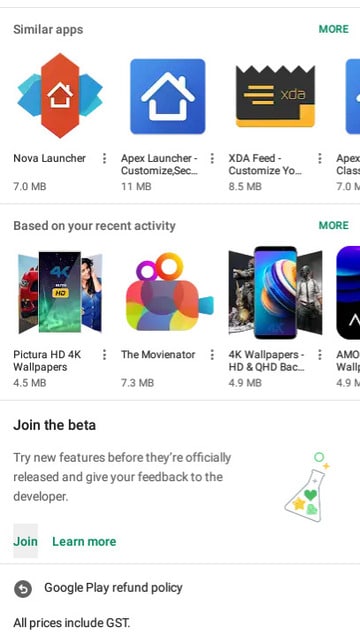The image showcases a selection of similar apps and recent activity apps on a mobile device screen. 

At the top, the similar apps are listed as follows:
1. **Nova Lounger** - Sized at 7.0 MB
2. **Apex Lounger Customize** - Sized at 11 MB
3. **XDA Feed Customize** - Sized at 8.5 MB

(Note: There is another app listed that is cut off and not visible.)

The second set of apps falls under a section labeled "Based on your recent activity," and the apps are:
1. **Picture HD 4K Wallpapers** - Sized at 4.5 MB
2. **The MovieNator** - Sized at 7.3 MB
3. **4K Wallpapers HD and QHD** - Sized at 4.9 MB

(Note: Another app is listed but is cut off and not visible.)

Below these apps, bold text reads: "Join the Beta. Try new features before they are officially released and give your feedback to the developer." Accompanied by a button icon reminiscent of a chemical laboratory item merged with a star and a heart, the section features options labeled "Join" and "Learn More" at the bottom.

Additionally, the image includes a Google Play refund policy disclaimer and states, "All prices include GST."